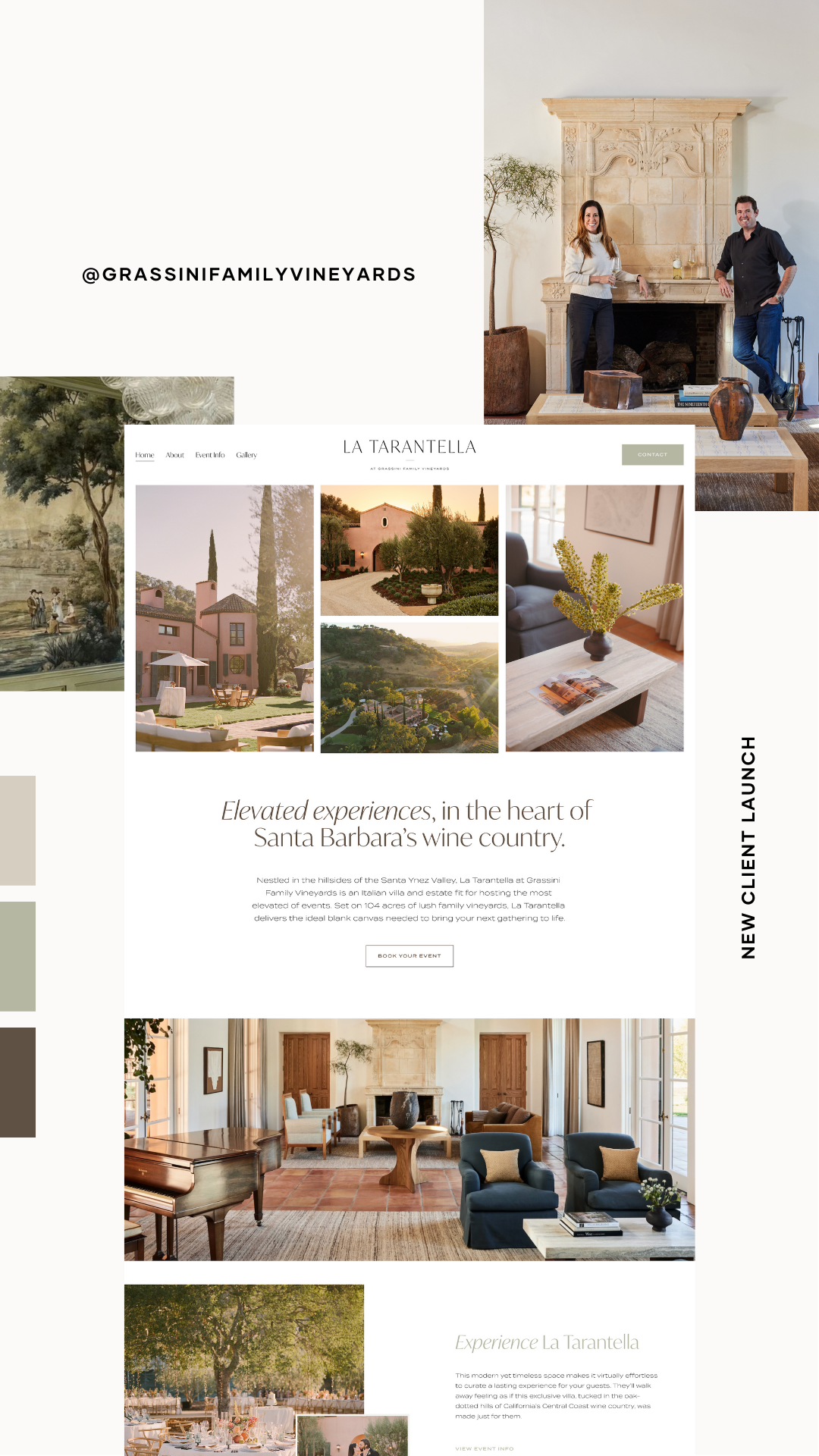This is a detailed description of a webpage designed for Grassini Family Vineyards. The webpage features a sophisticated layout with an artistic blend of overlapping images and text boxes. In the upper left corner, there's a simple white box displaying "Grassini Family Vineyards" in a single, continuous word. The page is adorned with numerous images of an elegant, stately home, suggesting the presence of a winery that might also function as a hotel, given the focus on luxurious rooms and scenic views rather than on wine itself.

On the lower right, a box extends upwards covering about two-thirds of the right-hand side, bearing the words "New Client Launch," hinting that this webpage might be a portfolio piece from a designer showcasing their work for Grassini Family Vineyards.

Additionally, there is a photograph featuring two individuals in front of a grand fireplace. The page also includes what appears to be an advertisement or flyer for another establishment, La Tarantella, which boasts "elevated experiences in the heart of Santa Barbara's wine country." The ad includes a brief, unreadable text segment, accompanied by a few pictures of La Tarantella, and a headline urging visitors to "Experience La Tarantella," followed by another paragraph of text.

On the left-hand edge of the page, three color swatches are visible, likely serving as test prints to ensure proper color density in the printing process. This detail further suggests that the webpage may be part of a broader design or promotional portfolio.